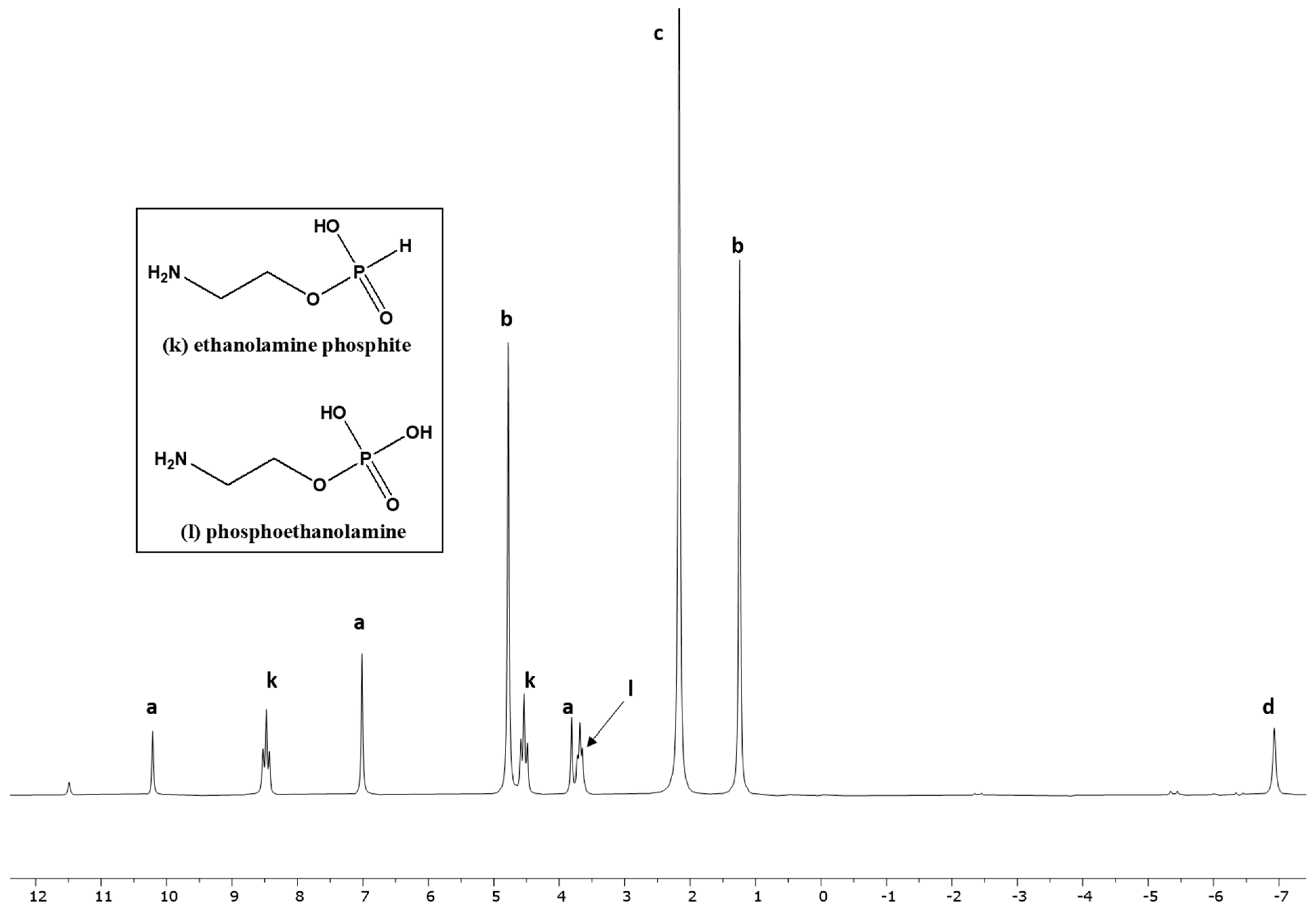The image depicts a detailed chromatogram with a solid white background featuring black text, graph bars, and key elements. On the top left, there's a square box containing the chemical structures of ethanolamine, phosphite, and phosphoethanolamine, the latter distinguished by an additional oxygen atom. Below this, the chromatogram exhibits labeled peaks of varying heights. The peaks are identified in sequence from left to right as A, K, A, B, K, A, I, C, B, and D. The horizontal axis, presumably representing time, is numerically marked from 12 down to -7, with negative values included. The overall layout and style of the graph are typical of those found in scientific publications, illustrating both the chemical compounds and their respective chromatographic profiles.